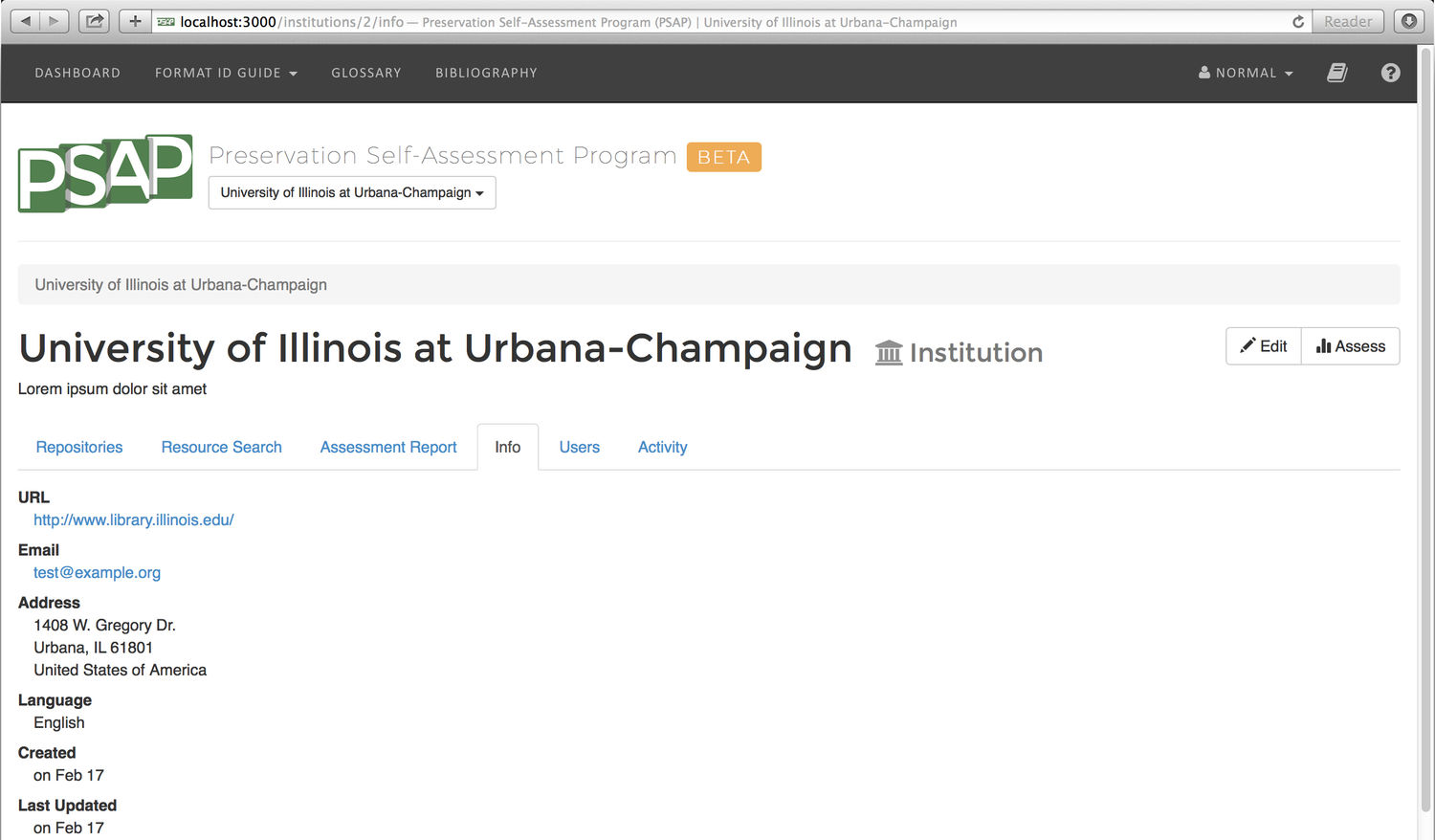This is a detailed screenshot of a web interface accessed locally at "localhost:3000", reflecting a testing environment. The top section features a gray bar displaying the URL address. Below it, a black navigation bar spans the width of the page, with menu options such as "Dashboard," "Format ID Guide," "Glossary," and "Bibliography" aligned to the left. On the right side of this bar, there is an option labeled "Normal" with a drop-down menu, accompanied by icons of two pages and a question mark.

Beneath the navigation bar, the bold heading "PSAP" is prominently displayed in white text set within green squares. Adjacent to "PSAP," the phrase "Preservation Self-Assessment Program" is featured, followed by an orange box labeled "Beta." Below this, the text "University of Illinois Urbana Campaign" is repeated twice, first as a singular line and then again above a large heading stating "University of Illinois at Urbana Campaign" alongside the word "Institution."

To the far right is a section with buttons labeled "Edit" and "Assess." Underneath, a series of selectable tabs include "Repositories," "Resource Search," "Assessment Report," "Info," "Users," and "Activity," with the "Info" tab selected. The detailed information presented under this tab includes:

- URL: http://www.library.illinois.edu
- Email: test@example.org
- Address: 1408 West Gregory Drive, Urbana, IL 61801
- Language: English
- Created on: February 17th
- Last updated on: February 17th